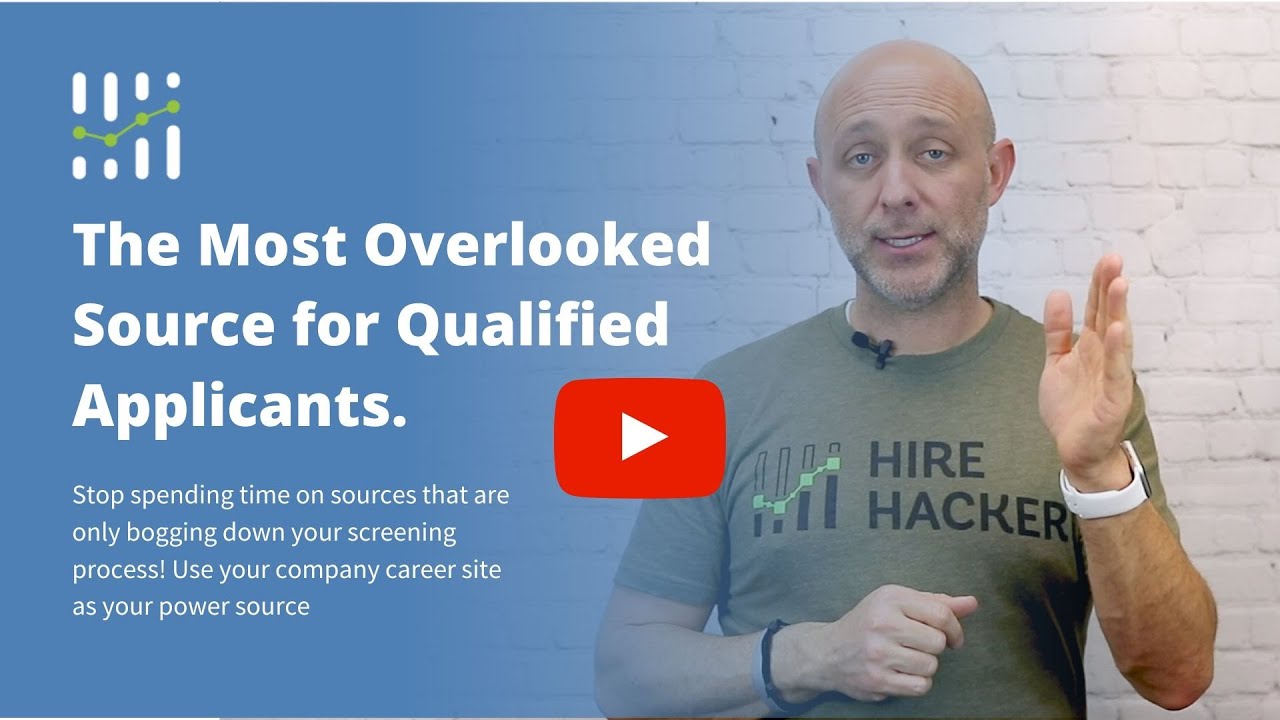A video thumbnail screenshot features a prominent red and white YouTube play button in the center against a blue background. On the left side, a green stock market trend line with bullet points intersects four vertical white lines. Below this graphic, the bold text reads, "The Most Overlooked Source for Qualified Applicants," with a subtext that says, "Stop spending time on sources that are only bogging down your screening process. Use your company career site as your power source." On the right, an older bald man with a graying mustache and closely cropped beard is facing the camera. He is wearing a khaki green t-shirt labeled "Hire Hacker" in black, along with the vertical line logo. The man has a white wristband, likely from an Apple Watch, on his left wrist, which is raised. His right wrist has a black band and is positioned near his abdomen. A black microphone is clipped to the neck of his t-shirt just below his chin.